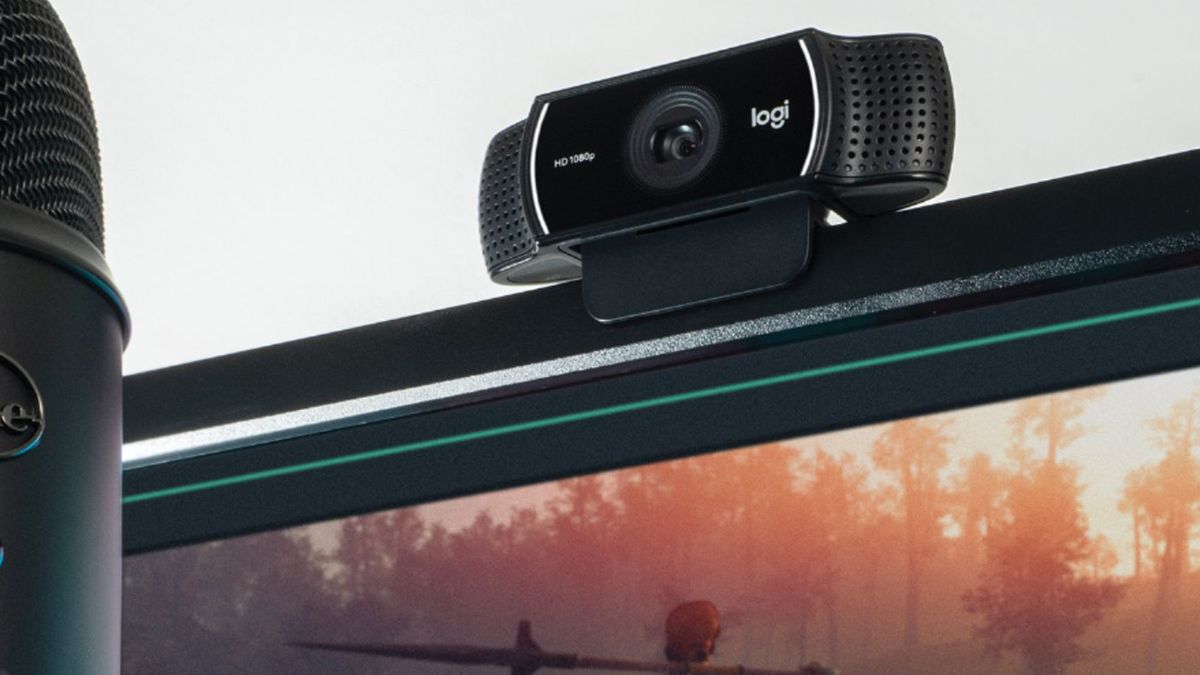This image features a black monitor displaying a picturesque sunrise or sunset, with sunlight streaming through a tree line and illuminating the scene. The monitor also depicts the edge of a helicopter rotor. Positioned at the center top of the monitor is a black webcam labeled "Logi" on the right and "HD 1080p" on the left, indicating its high-definition capability. The webcam appears to be clipped onto the monitor. Partially visible on the left side of the image is a black microphone, with a silver logo partially cut off. The entire setup, including the monitor, webcam, and microphone, seems geared towards enhancing computer-based video communication or streaming, capturing both the stunning on-screen scenery and the technical components in great detail.